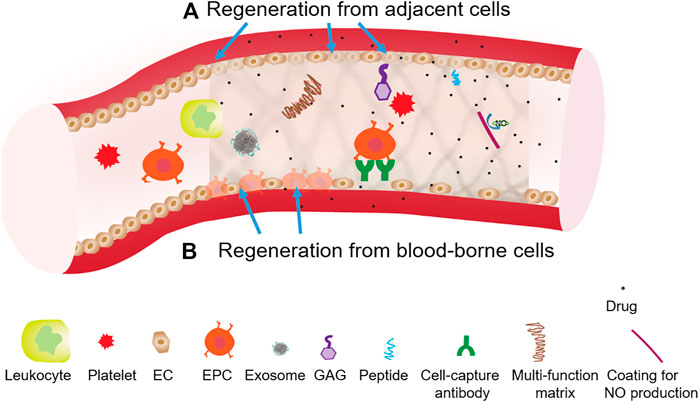The image is a detailed medical diagram divided into two sections. At the top, labeled "A," it illustrates "regeneration from adjacent cells" with an arrow pointing to various cells of different colors: red, orange, yellow, and blue. Beneath this, labeled "B," it depicts "regeneration from blood-borne cells" with several blue arrows pointing at different blood cells surrounded by a red outer wall resembling a vein or tubing. 

The diagram highlights various elements, each labeled precisely. The legend at the bottom identifies these elements:
- A red circle with a squiggly line for "multifunction matrix"
- A yellow blob with a green amorphous shape for "leukocyte"
- A spiky red circle for "platelet"
- An orange circle marked "EC"
- An orange circle with four protrusions for "EPC"
- A gray blob for "exosome"
- A purple hexagon for "GAG" with a single hook
- A blue squiggle for "peptide"
- A green three-armed symbol for "cell capture antibody"
- Small black dots representing "drug," which has a purple line indicating "coding for no production"

The diagram effectively demonstrates different cellular components and processes involved in cell regeneration, with clear visual indicators and a corresponding legend for easy interpretation.